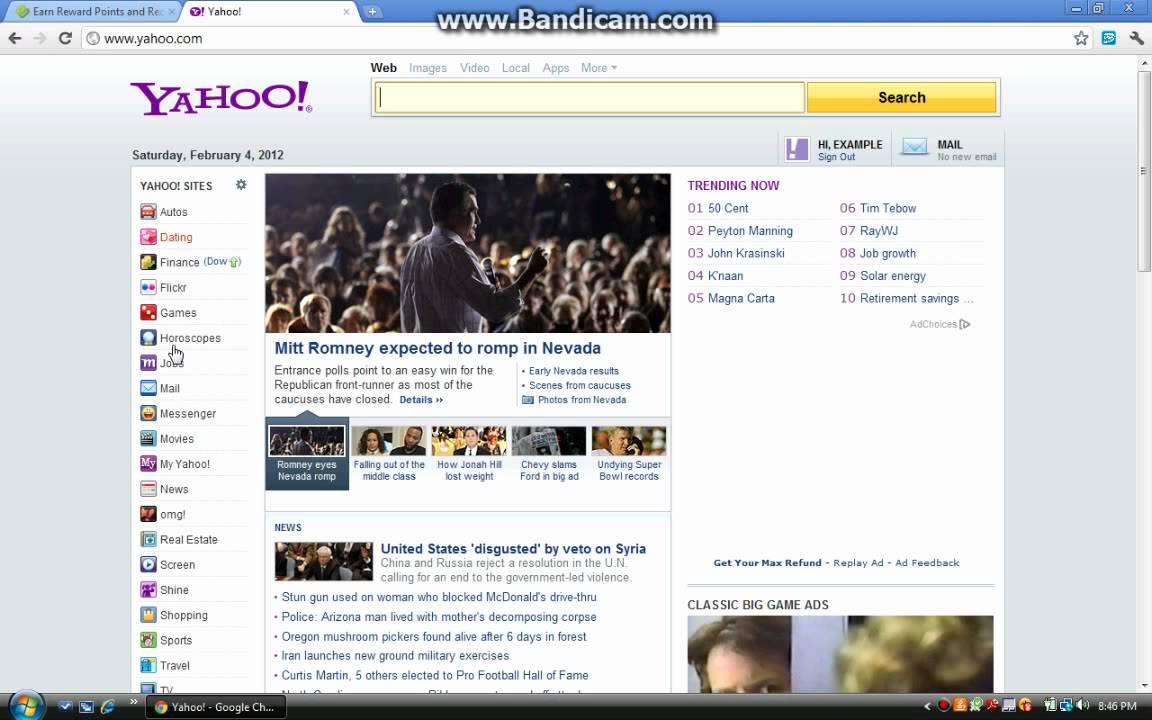This screenshot captures a Windows desktop screen displaying the Google Chrome browser with two open tabs. The active tab is navigated to Yahoo.com, as indicated by the URL in the address bar. At the top left corner, the purple Yahoo logo with an exclamation point is prominently visible. To the right of the logo, there's a yellow search bar accompanied by a yellow search button on its right side.

Above the search bar is a navigation menu containing six links: Web, Images, Video, Local, Apps, and More. On the left side of the page, there's a sidebar labeled "Yahoo Sites." The Windows taskbar is visible at the bottom of the screen, completing the classic desktop layout.